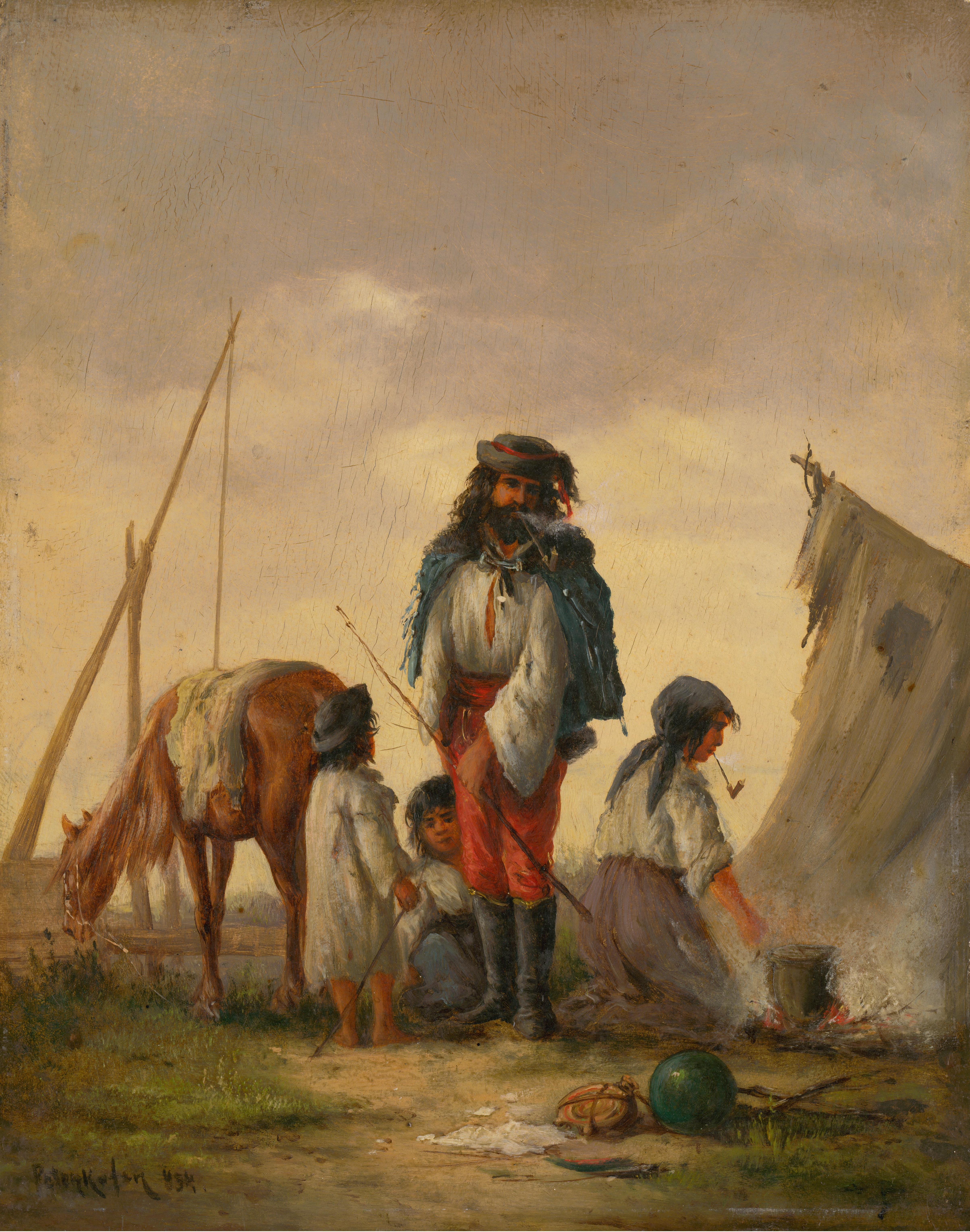The painting, set in a dusty and cloudy landscape evoking the Wild West era, depicts a tattered settler scene with a rugged family encampment. At the center stands a bearded man with long black hair, wearing a wide-brimmed hat adorned with a feather. He is dressed in a white button-down shirt with wide sleeves, red pants tucked into tall black boots, and a tattered blue cape or animal fur draped over his shoulders. The man is holding a fishing pole and smoking a pipe. In the foreground, there are two children in dirty white gowns; one is standing, while the other sits on the ground behind him. To the side, a brown horse with a blanket over its back grazes nearby. A woman, potentially the man's wife, is kneeling at a campfire with a smoking corn pipe in her mouth. She wears a long dark blue skirt, a light blue or white shirt, and a blue rag tied around her head. The encampment includes a small, ragged tent, a blue or green ball, a broken water canteen, and a spilled white substance on the ground, all on a patch of green grass. The overall tone of the painting is gray and beige, with hazy clouds, creating a sense of both ruggedness and nostalgia.